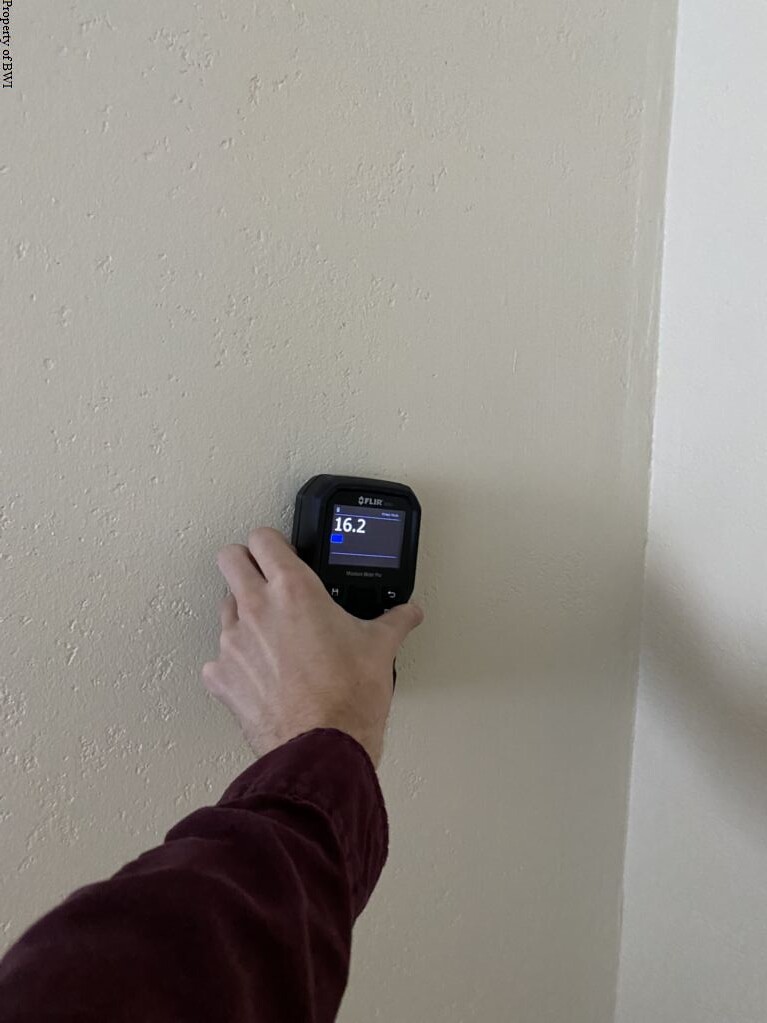This rectangular, vertically-oriented photograph centers around a white stucco-textured wall, captured with great attention to detail. The wall, making up the majority of the background and occupying approximately four-fifths of the image, intersects with a slightly lighter white wall at the corner. Emerging from the lower left corner of the image is a Caucasian hand, visible from just below the elbow. The hand, belonging to what appears to be a male, indicated by the slight body hair, is clad in a dark long-sleeved shirt or jacket. It is holding a black, handheld electronic device branded FLIR, which displays a digital readout of 16.2 in white text. The hand is firmly pressed against the creamy white wall, emphasizing the device's interaction with the surface. The intricate contrast of wall textures and subtle color variations, alongside the focus on the measuring device, creates a detailed and engaging composition.